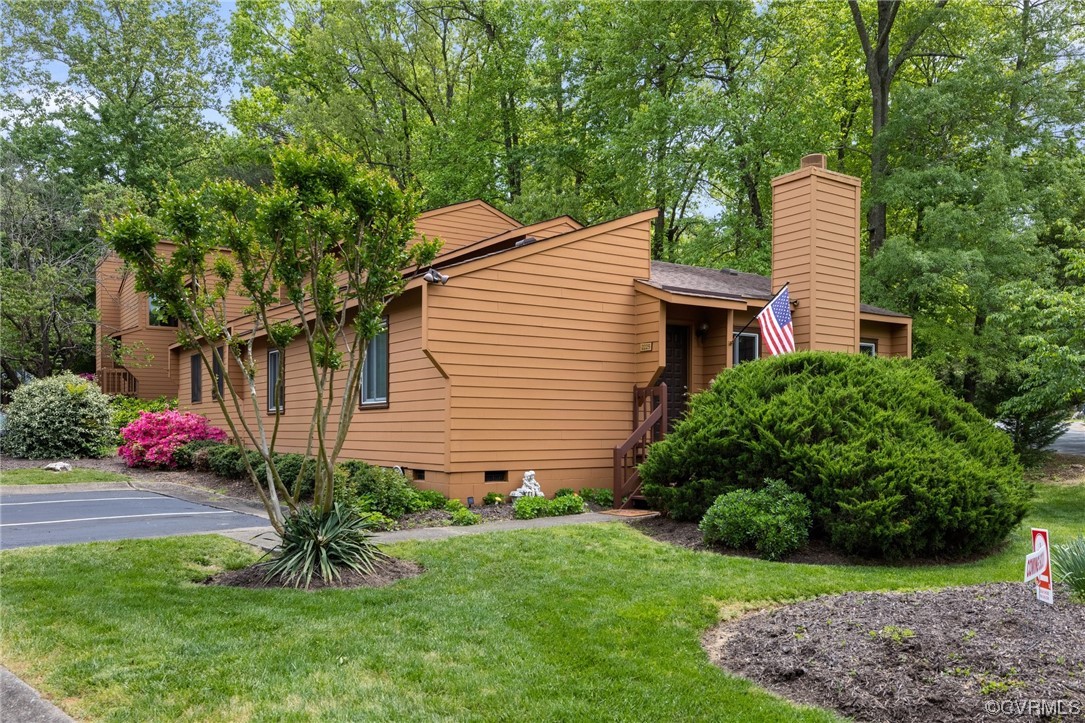This color photograph captures an exterior view of a residential building, possibly an apartment complex or townhouse, characterized by its brown horizontal lap siding and dark brown tiled roof. The building has a striking geometric roof plan and features an American flag hanging on a post near a small porch with a handrail leading up to the doorway. The complex includes multiple units, with some being single-story and at least one two-story unit, as indicated by the chimneys and varied roof elevations.

The landscaping in front of the building is meticulously maintained, featuring a freshly cut lawn with some dry patches. Prominent in the foreground is a large, round shrub and a blooming pink azalea bush, along with a larger shrub with white flowers. There are several other smaller bushes and a mound of junipers, alongside a low hedge and possibly an aloe plant. The layout is further accentuated by mulch garden beds and a crepe myrtle tree toward the left.

The scene includes two designated parking spaces marked by white stripes in front of the building, suggesting this is a multifamily residence. A realtor or promotional sign is visible in one of the garden beds, though the text is unreadable.

Background elements include a dense array of green trees that frame the building, adding depth and indicating a forested area behind the complex. The overall atmosphere is complemented by a clear, blue sky, pointing to a serene day, likely in springtime, given the blooming flowers.